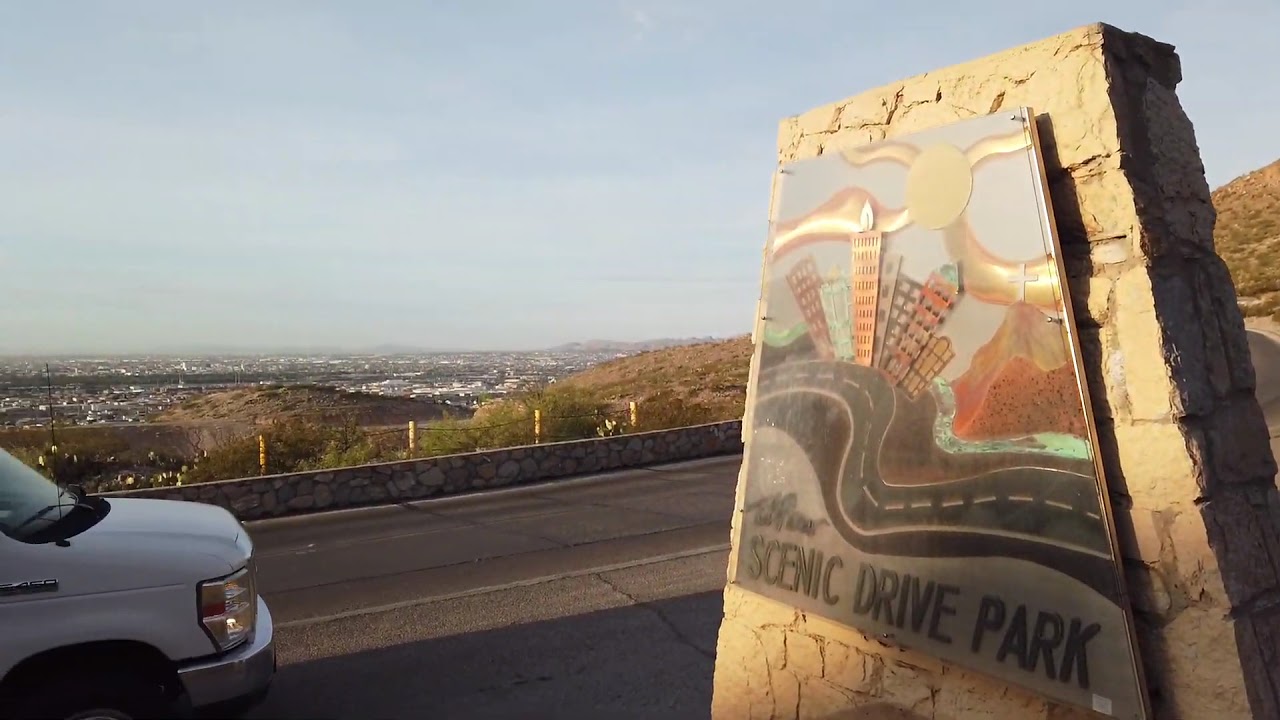The image captures a scenic overlook, focusing on a stone sign on the right which reads "Scenic Drive Park." The sign features a 2D illustration of a winding street with skyscrapers, a sun in the sky, and a cross on a hill, set in a distinctive pentagon-like, cream-colored cement and brick structure with a glass frame on top. The foreground shows a black asphalt road and a large sidewalk bordered by a brick wall. The bottom left of the image includes the hood of a white van. In the background, a sprawling cityscape with numerous buildings and white rooftops extends into the distance under a partially cloudy, light blue sky.